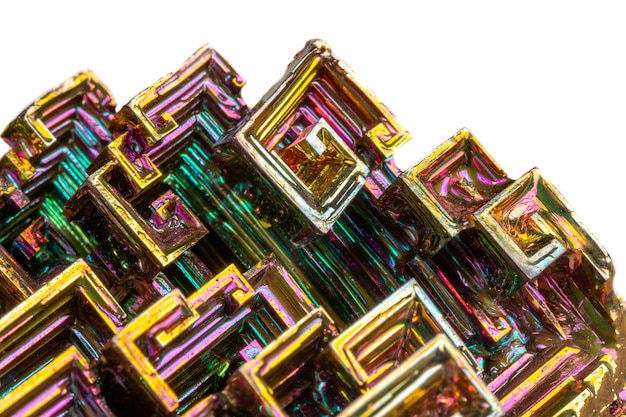The image depicts an abstract, multicolored geometric structure against a white background. The structure, which covers the bottom two-thirds of the frame, appears to be composed of a variety of conjoined square and T-shaped elements that create a complex, layered composition. The object has a reflective, metallic surface that exhibits a spectrum of colors, including prominent shades of magenta pink, green, blue, teal, gold, purple, yellow, aqua blue, and orange. Its intricate design features a combination of gemstone-like and skull-like metallic rims which enhance its abstract, almost otherworldly appearance. The precise nature of the object is unclear, lending it an enigmatic and interpretative quality, highlighted by greenish and reflective shadows that add to its depth and complexity.